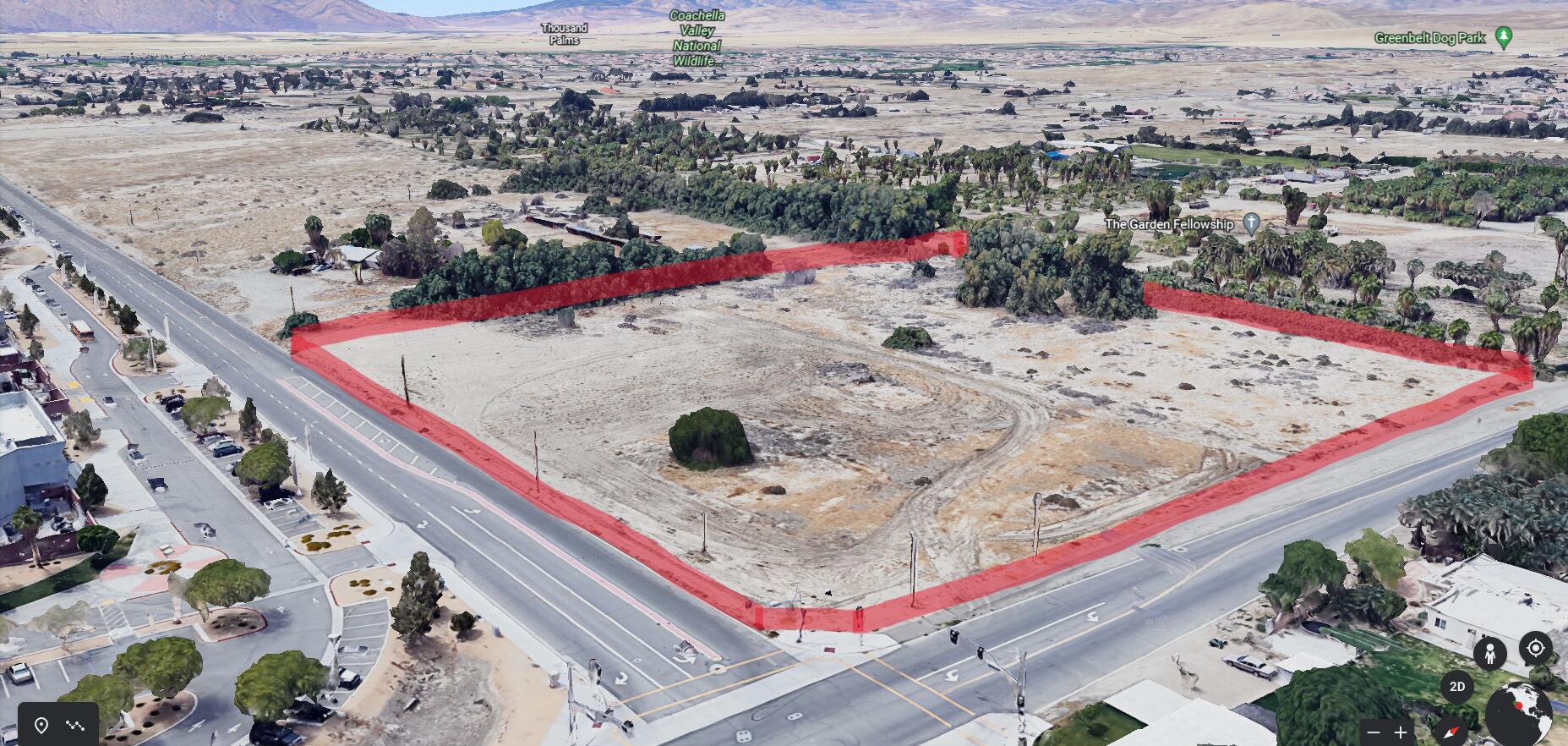The aerial view captures an empty lot outlined with a red highlight, indicating its boundaries. The undeveloped lot features dirt terrain interspersed with small shrubs and a few larger ones concentrated towards the back. The immediate surroundings are sparse, populated with more green vegetation, including bushes and trees. The lower sections of the image reveal several roadway cross sections, with buildings and parked cars visible in parking lots toward the bottom left. A trail or road runs through the center of the lot, suggesting some usage or passage through this otherwise barren land.